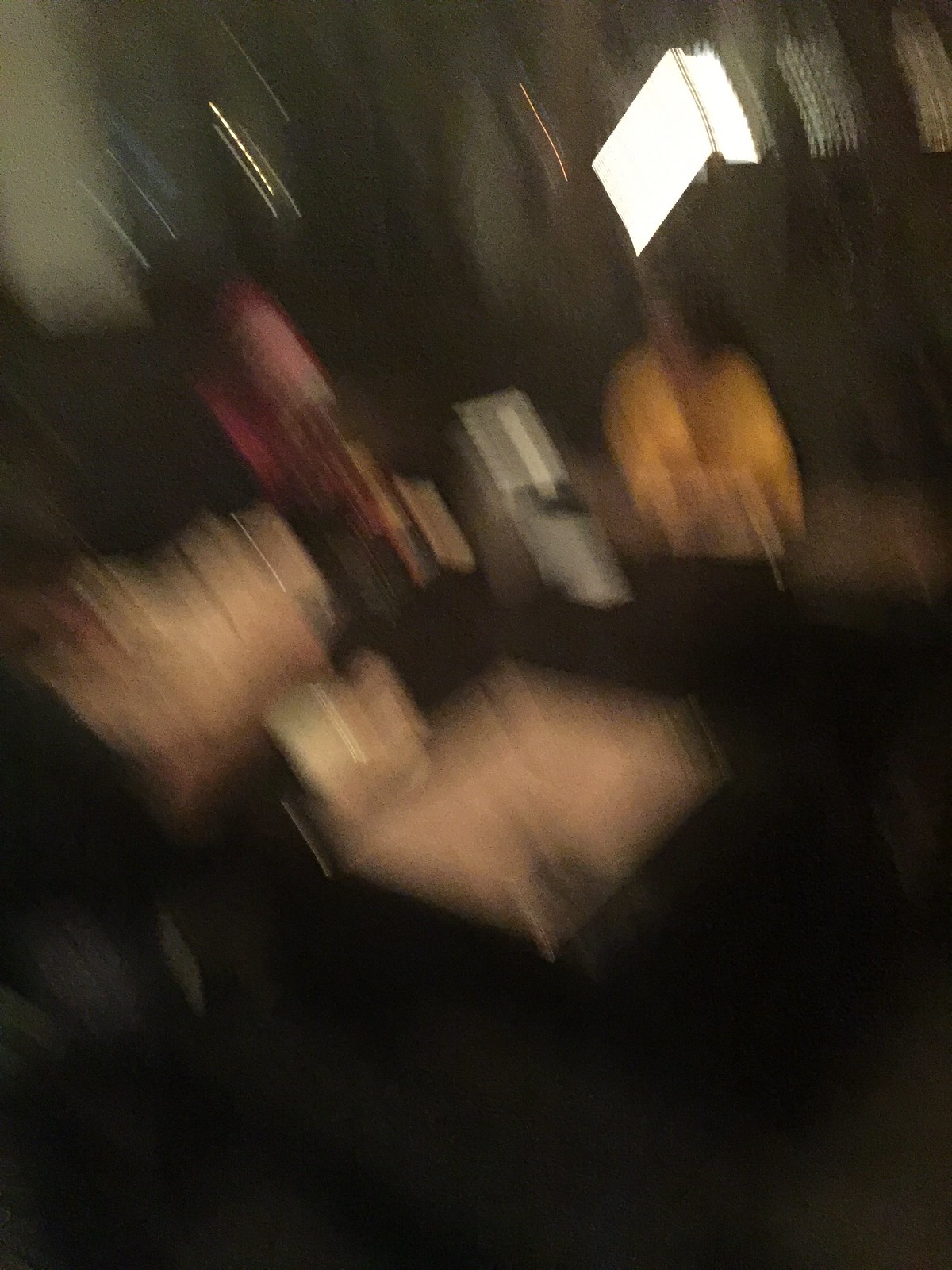In this very blurry nighttime photograph, the composition features a scene with various points of interest. Toward the upper right corner, a rectangular light source is captured at a diagonal angle, contributing to the ambient illumination. Below this light, a woman stands prominently, dressed in a striking yellow V-neck dress. Her dark hair cascades around her as she turns slightly to her left, suggesting movement or a candid moment. She appears to be positioned near a desk or bar, which is adorned with a collection of glasses and a bottle of wine or champagne, indicating a festive or social setting. The background features thin white lines of light scattered throughout, adding to the overall atmosphere. The upper left portion of the image is clouded, and the bottom section fades into complete darkness, framing the scene in a contrasting manner.